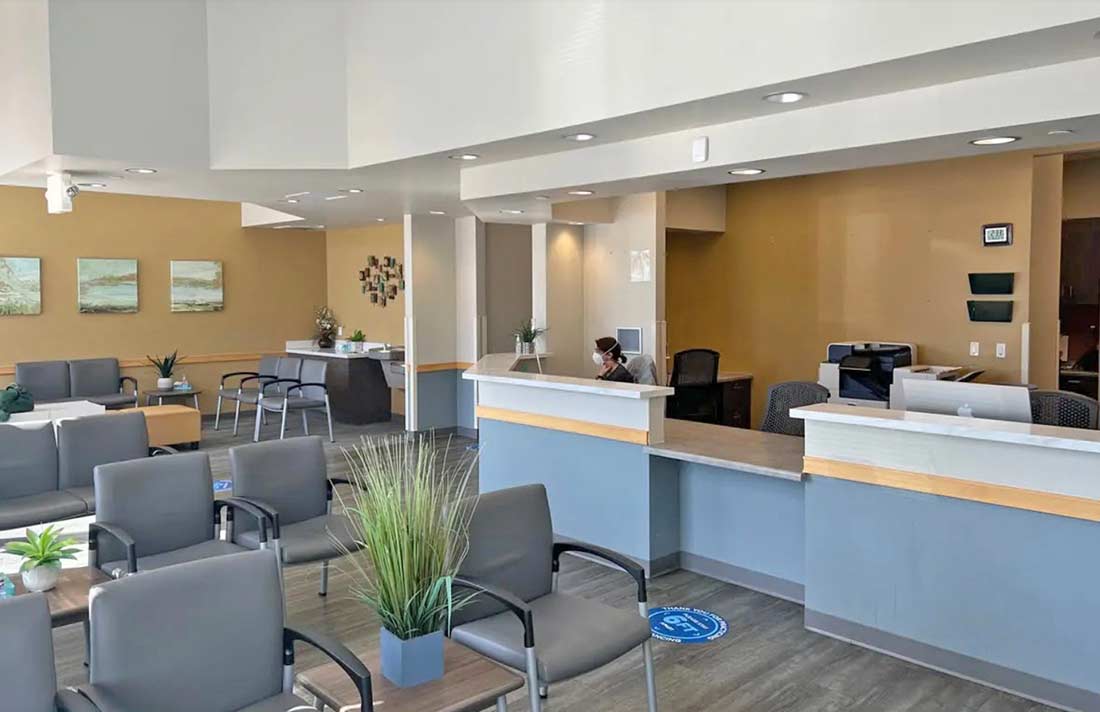The image portrays a reception area of a medical office. A counter with an open section allows for the exchange of documents; a woman, likely a receptionist, sits behind it wearing a medical mask and holding one hand on her neck. She appears to be working at a computer, with a printer visible behind her. The waiting room is furnished with numerous gray chairs featuring black armrests, and the space is adorned with potted plants, whose authenticity is uncertain. The ceiling is white with recessed lighting, and the top of an Apple Macintosh monitor is visible, adding a touch of modern technology to the setting.